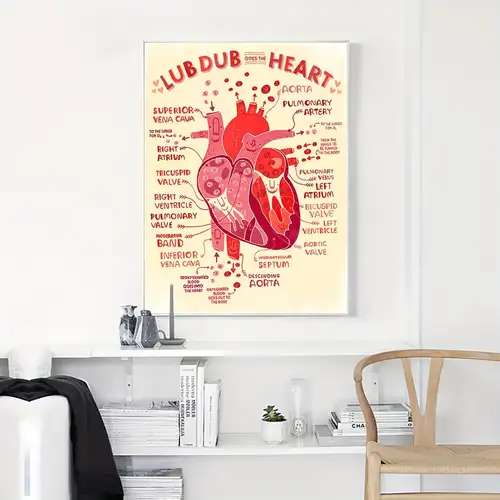The photograph captures a minimalist-themed room dominated by white hues. A large poster, illustrating a colorful and whimsical anatomical diagram of a human heart, is prominently displayed on a white wall. The poster, which is titled "Lub Dub Goes the Heart," merges scientific details with playful elements, featuring labels for parts of the heart such as the aorta and superior vena cava, and is adorned with small heart icons in shades of red, dark magenta, bright cherry red, rosy pink, and cream.

Below this vibrant poster stands a low white bookcase. On its multiple layers, which serve as both shelves and surfaces, stand white hardback books, stacks of magazines or paperback books with white covers, a white flower pot containing a small green plant, a white candlestick, and various figurines. Situated to the right of the bookcase is a light brown, or beige, wooden chair facing the viewer, characterized by a bent wood design and open back. Adding a slight contrast, a white object with a black coat draped over it is visible on the left side of the image. The overall aesthetic is clean, minimalistic, and sleek, with the poster providing the primary burst of color in the room.